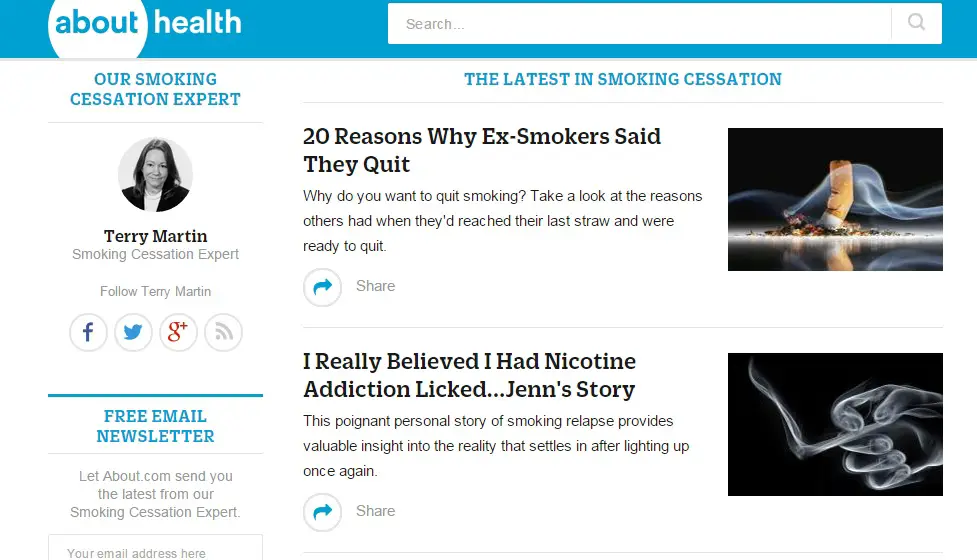**Descriptive Caption:**

In this informative screenshot from a health website, the title "About Health" is prominently displayed in the top left corner, while a search bar is conveniently located at the top right. The left sidebar features an introduction to Terry Martin, identified as the Smoking Cessation Expert, along with links to follow Terry Martin on Facebook, Twitter, and Google Plus. It also highlights an option to subscribe to a free email newsletter provided by Letabout.com, designed to keep readers updated with the latest insights from the Smoking Cessation Expert.

The main content introduces a section titled "The latest in smoking cessation," featuring an article, "20 Reasons Why Ex-Smokers Said They Quit." This piece invites readers to explore the motivations behind others' decisions to quit smoking and encourages them to share their own reasons for quitting.

Adjacent to this text is a striking photograph depicting a cigarette stubbed out in a pile of ash, with tendrils of smoke delicately swirling around the extinguished cigarette butt. Below this, another poignant story is shared: "I Really Believed I Had Nicotine Addiction Licked, Jen's Story." This personal narrative offers a compelling look into the challenges of smoking relapse and the harsh realities faced after resuming smoking. Readers are once again encouraged to share their thoughts.

To the far right is a visually captivating photo illustration. It artistically portrays a hand holding a cigarette, both crafted from smoke, with delicate wisps forming the hand and cigarette butt, emphasizing the ethereal and fleeting nature of smoking.